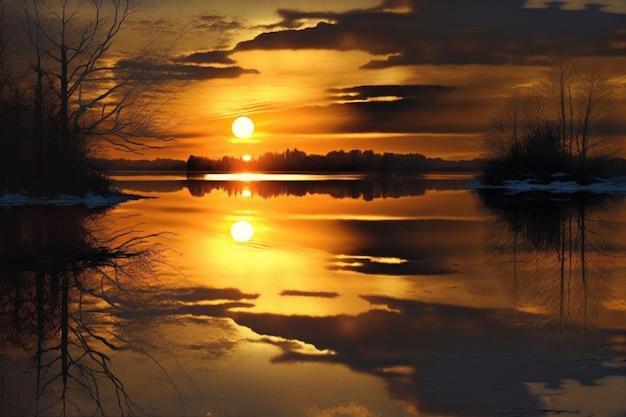This is a highly detailed photograph of a stunning sunset over a large, tranquil lake with portions of the water frozen. The sky is painted gold by the setting sun, which is haloed in orange. The sun sits just above the horizon, casting a white light with an orange glow that seamlessly reflects on the calm, glass-like surface of the lake. Parts of the water exhibit a frosted look, suggesting ice patches that differentiate from the liquid areas. The reflection of the sun, along with the dark silhouettes of leafless trees on both the left and the right, mirrors perfectly in the water below. The horizon is positioned toward the upper third of the image, emphasizing the vast expanse of the lake and the sky.

Several islands are present, scattered across the lake and covered in black, skeletal trees, indicating a winter season. Some islands have hints of snow, adding to the wintry ambiance. Dark clouds, both brownish and reddish, hover above and are mirrored below, further enhancing the symmetry. Near the center, the bright yellow sun forms a distinct beam across the sky and water. On the left, a significant tree stretches to the top left corner, while similar leafless and evergreen trees occupy the right side. The serene and almost pristine reflection of the trees, sky, and clouds on the lake's surface gives the composition a deep, almost surreal quality, making it difficult to discern if the image is a photograph or digital artwork.